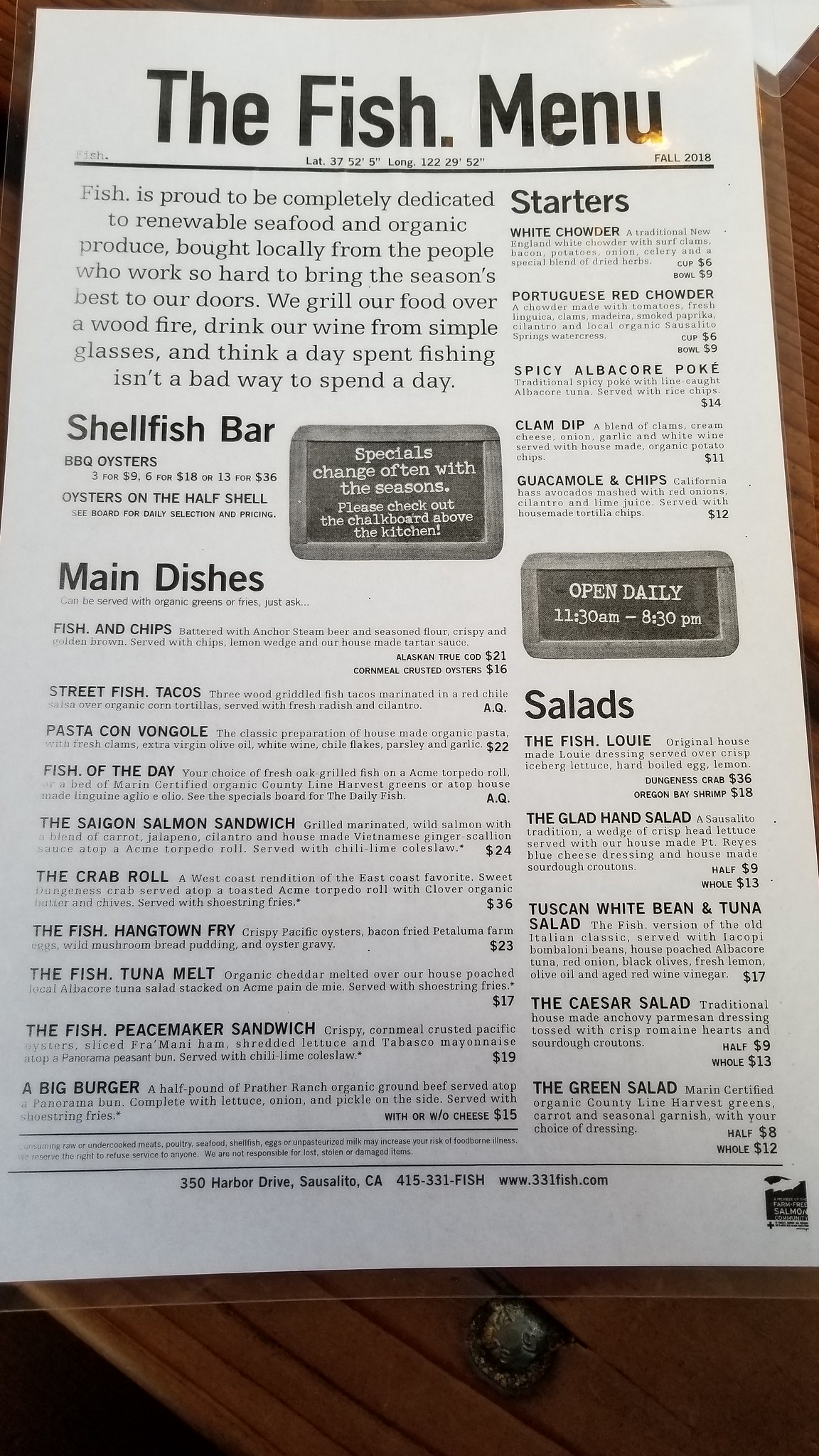In this indoor digital photograph, the upper right corner features a laminated white menu, shielded by a clear plastic cover. The bottom left of the image is notably dark, revealing a section of a darker wooden table, held steady by a conspicuous, rusty silver bolt. Dominating the central portion of the photo is another white laminated menu, emblazoned with bold black text. The large heading reads "Fish Menu." Below, the coordinates of the restaurant's location are neatly printed. 

To the left side of the menu, the text “Fall 2018” is outlined above a thick black line, introducing the main body of the menu. The descriptive passage proudly states: "Fish is proud to completely dedicate the renewal of seafood and organic produce brought locally from the people who work so hard to bring the season's best to our doors. We grill our food over a wood fire, drink our wine from simple glasses, and think a day spent fishing isn't a bad way to spend the day."

Beneath this text, the menu is organized into sections like "Shellfish Bar" in prominent print, detailing the available choices. Further to the right, at the top, it says "Starters," followed by the restaurant's operational hours, listed as 11:30 AM to 8:30 PM daily. Below this, another section labeled "Salads" appears. At the bottom of the page, the location of the restaurant and its website are provided. The bottom right corner features a striking black logo, further solidifying the menu's polished and professional appearance.